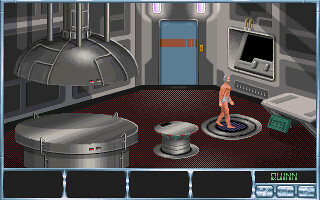This image is a detailed screenshot from the point-and-click adventure video game *Return to Ringworld*. Set in a futuristic room that resembles a control room on a spaceship, the scene is primarily gray with metallic walls and a maroon-colored floor. The room features an octagonal shape with a mix of oval elements and cylindrical metal equipment. Dominating the background is a blue door adorned with an orange stripe and flanked by two lights overhead. The door's opening mechanism appears to be a small yellow square with an orange button in the center.

In the middle of the room, there are two circular platforms, including a silver circle on a movable pole that emerges from the central circle on the ground. Also present is a screen and a white table. The character in mid-step, likely named Quinn, is moving across the room. He is identifiable by his orange jumpsuit, which was mistakenly described as gray shorts or underwear, and is characterized by his gray hair and beard. Along the bottom of the image, there are five rectangles and a numeric "three" in the right-hand corner, indicating aspects of the game's interface or HUD elements.